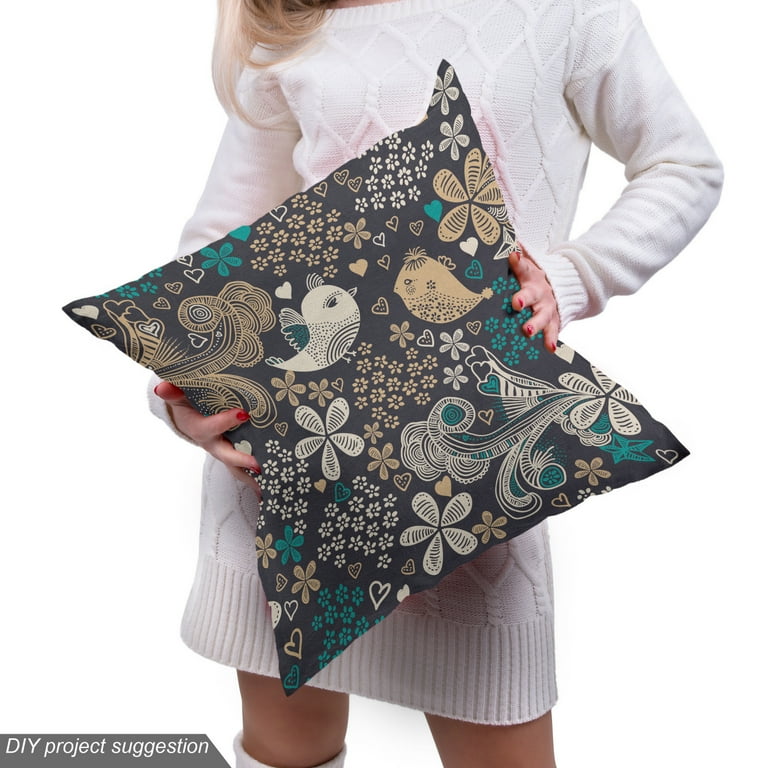The image features a white background with a "DIY Project Suggestion" banner in the bottom left corner. Central to the photo is a woman, shown from the neck down, wearing a white long-sleeved sweater dress that extends to her knees. She has fair, Caucasian skin and red nail polish. The woman is holding a dark gray square pillow at an angle, decorated with floral designs in teal, white, and beige hues. The pillow also features images of two birds, one white and one yellow. The intricate design includes abstract patterns with hearts and stars in muted colors. Visible at the bottom of the image, the woman appears to be wearing white boots or high socks on one leg.